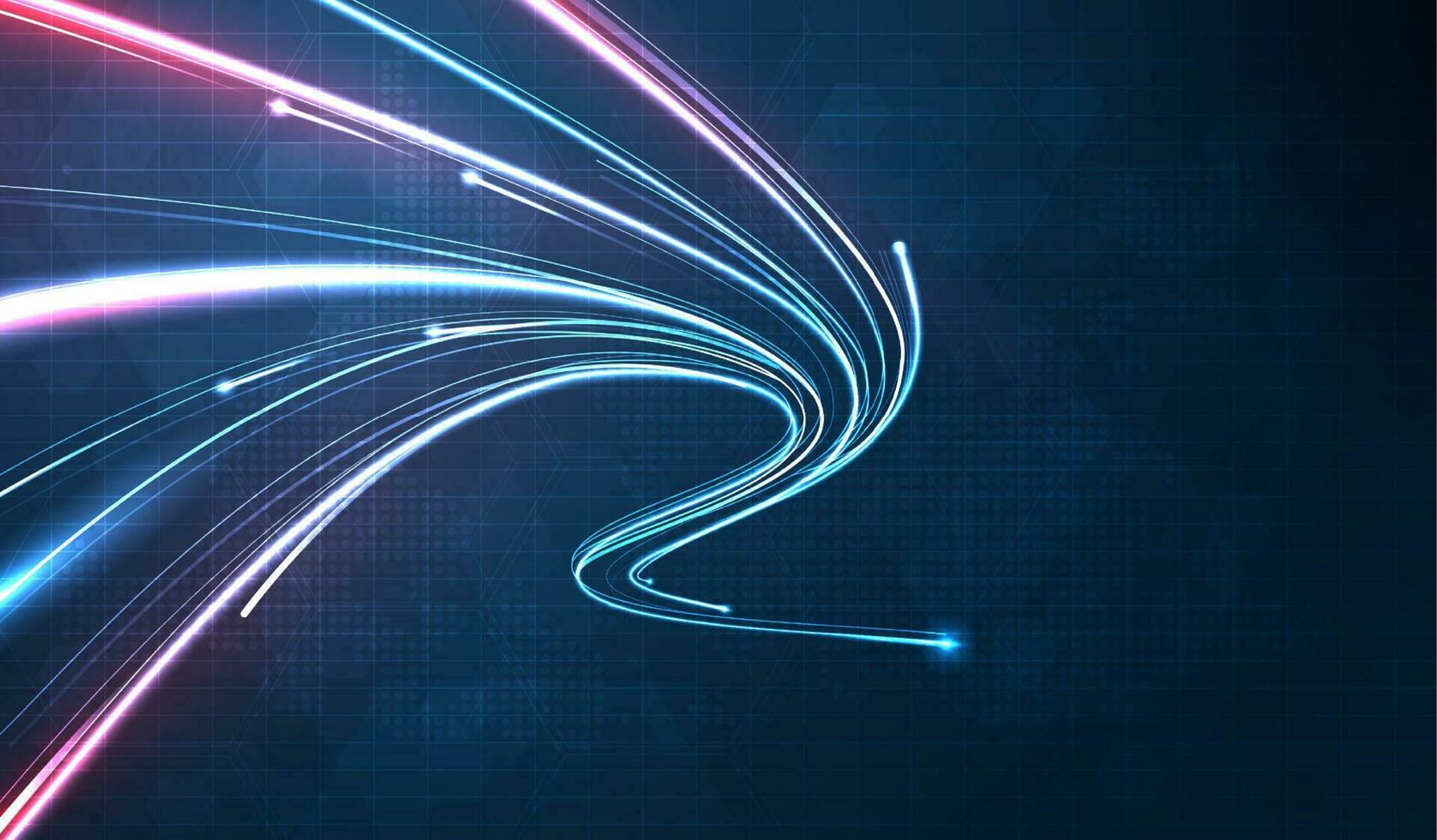The image is a piece of digital art with a striking and intricate composition. The background is a gradient of dark to light blue, featuring faint, grid-like lines intersecting to form subtle rectangular patterns. Additionally, there are faded hexagonal shapes interspersed within the background, adding a layer of complexity. The right side of the image transitions into a dark, almost black shade.

At the lower center of the image, a bright light emerges and swirls upward, forming an S-shaped pattern that extends left and right before fanning out. This swirling light comprises approximately 10 to 15 vibrant lines in varying thicknesses and colors, including neon purples, blues, teals, pinks, and whites. These lines exhibit a gradient effect, transitioning seamlessly from one color to another, and enhance the image's dynamic feel. At the tip of each curve in the S-shape, a prominent bright light or "head" appears, emphasizing the movement and flow of the lines. Overall, this intricate and vibrant display creates a stunning visual of light and color in motion against a high-tech, digital background.